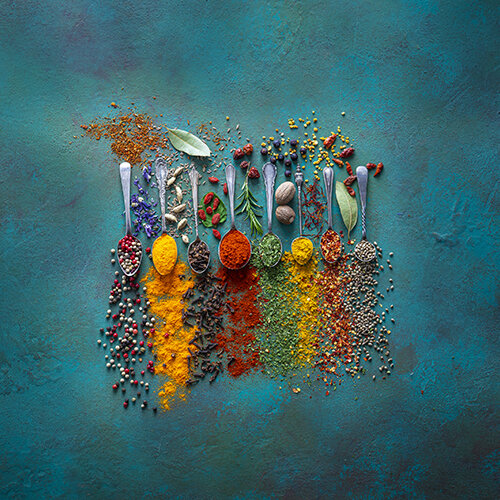This vivid photograph captures a striking top-down view of eight spoons meticulously arranged in a straight horizontal row against a textured bluish-green background. Each spoon contains a colorful assortment of spices and food items, which are artfully spilled beneath them, creating vibrant trails that draw the eye downwards. Starting from the leftmost side, the first spoon holds round beads in red, white, and purple hues, with more scattered beneath it. Adjacent to it is a spoon filled with bright yellow turmeric, leaving a golden trail below. The third spoon contains dark and coarse material resembling chocolate shavings, while the fourth holds a vibrant orange spice, such as paprika, with rice-like grains sprinkled above. Moving right, the fifth spoon features a green, grainy substance with a pair of large white nuts lying between it and the adjacent utensil. The next spoon showcases yellow powder, trailed beneath, with a hint of green substance above. To its right, a spoon holds a mix of red and yellow grains, with a green leaf and a small red pepper between this spoon and the final utensil. The last spoon carries white and purple pellets, with a scattered trail below. Sprinkled herbs and vibrant green leaves are interspersed among the spoons, adding an additional layer of natural texture to the arrangement. This carefully composed image contrasts the bold colors of the spices against the cool, artistic teal backdrop, creating a feast for the eyes.